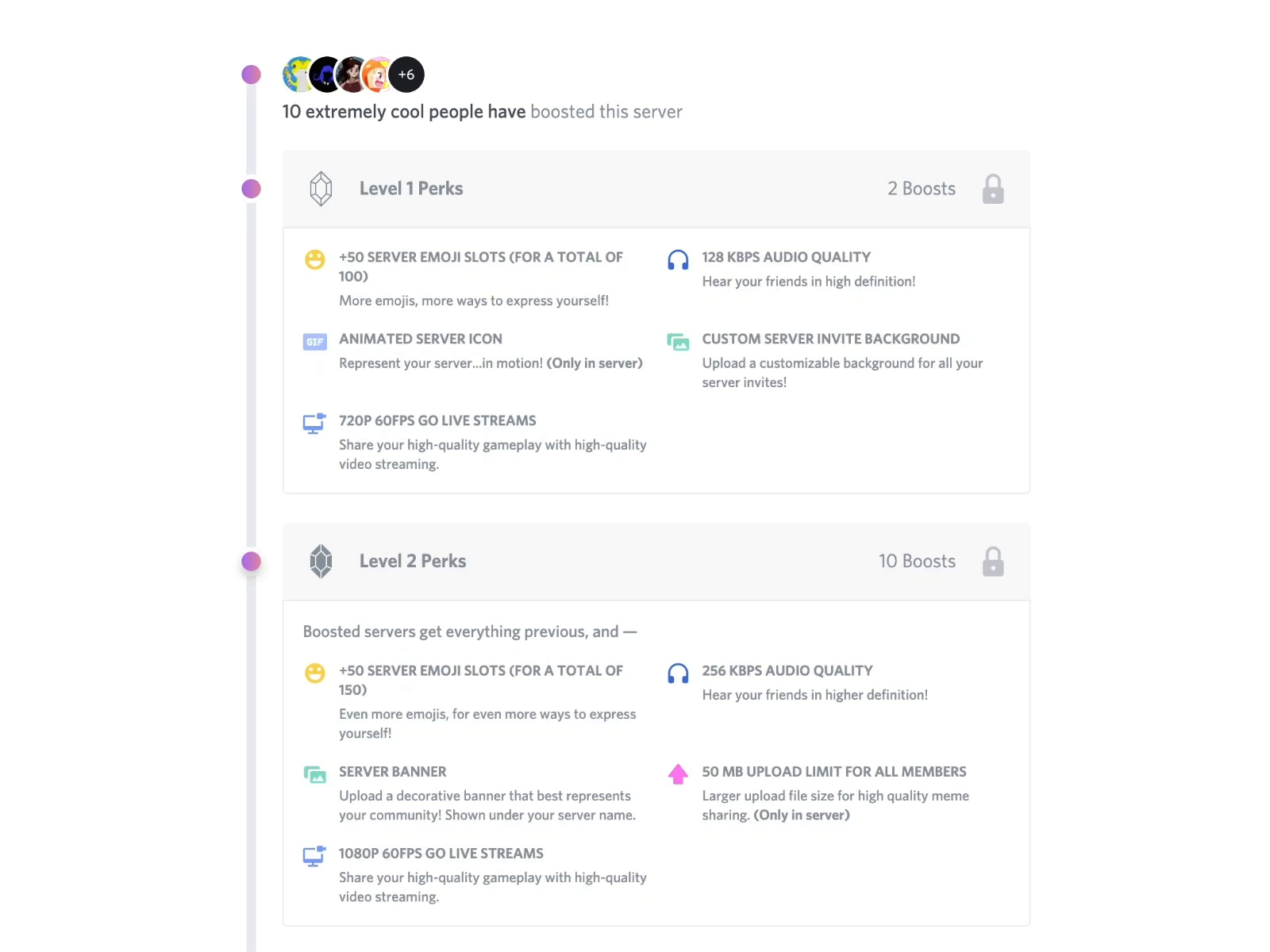This image is a screenshot from a website featuring a predominantly white background. On the left-hand side, a grey vertical line runs from the top to the bottom, punctuated by three purple dots. 

At the top of the image, next to the first purple dot, there's an array of profile picture circles followed by the text, "10 extremely cool people have boosted this server." Below that, adjacent to the second purple dot, is a pale grey block featuring a gem icon on its left side. Next to this icon, the text reads "Level 1 perks." Moving rightward from this block, there is a padlock icon and the text "2 boosts." Nearby, a yellow circular symbol is accompanied by the text "50 server emoji slots for a total of 100." Further down are icons representing additional perks: a blue icon for an animated server icon, a screen icon indicating "720p, 60fps, go live streams," a headphone symbol indicating "128kbps audio quality," and two green rectangles denoting a "custom server invite background."

The third purple dot, further down, corresponds with another pale grey block. This one contains a colored gem symbol and the text "Level 2 perks." To the right, it mentions "10 boosts" next to another padlock icon. Below, on a white background, it indicates "Boosted servers get everything previous and more." Listed perks include "50 server emoji slots," "server banner," "1080p, 60fps, go live streams," "256kbps audio quality," and the ability to upload files up to "50 MB for all members." 

The detailed icons and descriptions collectively outline the benefits and levels of server boosts, offering a clear view of potential upgrades and enhancements.